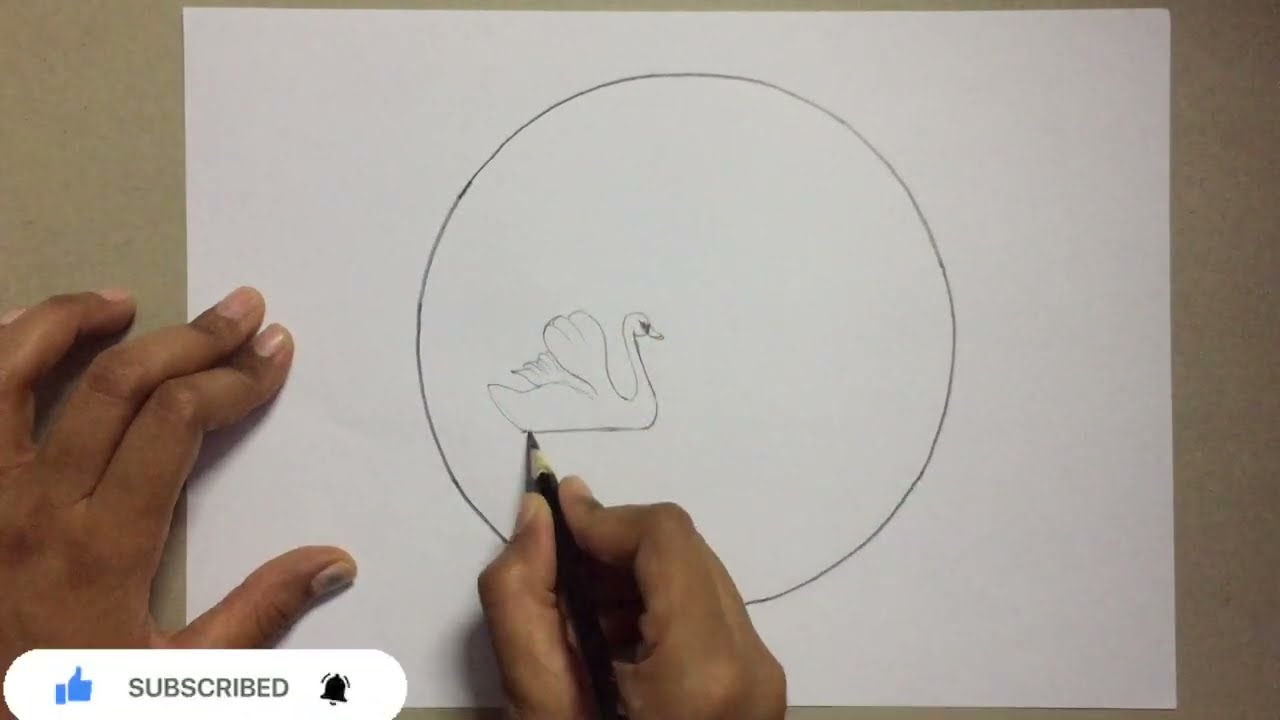The image is a top-down view of a white piece of printer paper in landscape orientation, taking up most of the frame. It seems to be a still from a YouTube video tutorial on drawing. In the center-left of the paper, there's a sketched circle within which a detailed, 2D profile of a swan is in progress. The swan, swimming from left to right, has its eyes, beak, and many feathers already outlined. The artist is currently working on the bottom part of the swan. Two hands are visible: the left hand, which is brown-skinned, holds the paper steady, while the right hand wields a black pencil for drawing. In the bottom-left corner of the image, there is a YouTube interface with a "Subscribed" status, a thumbs-up icon, and a ringing bell icon, indicating the video is part of a channel's instructional content.